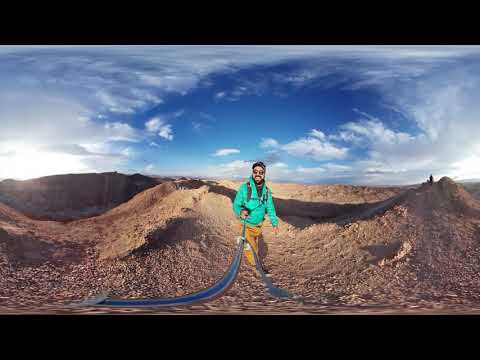In this surrealistic composition, a man stands prominently in the center, hiking through what appears to be a desert-like or mountainous terrain made up of brownish, rocky hills. He’s wearing a bright green jacket and yellow-orange pants, complemented by sunglasses, a hat, and a goatee. The distorted perspective shows him smiling and holding a blue selfie stick, which bends to form a wavy curve enhancing the surreal feel of the image. The sky behind him is striking, predominantly filled with billowing clouds that loop around to reveal a blue center, adding depth to the scene. To the left of the frame, a vibrant sunset or sunrise is captured just above the horizon, casting long shadows across the sandy or stony foreground. Faintly, to the right, the outline of another person appears, possibly hiking up a road, emphasizing the isolation and vastness of the landscape.